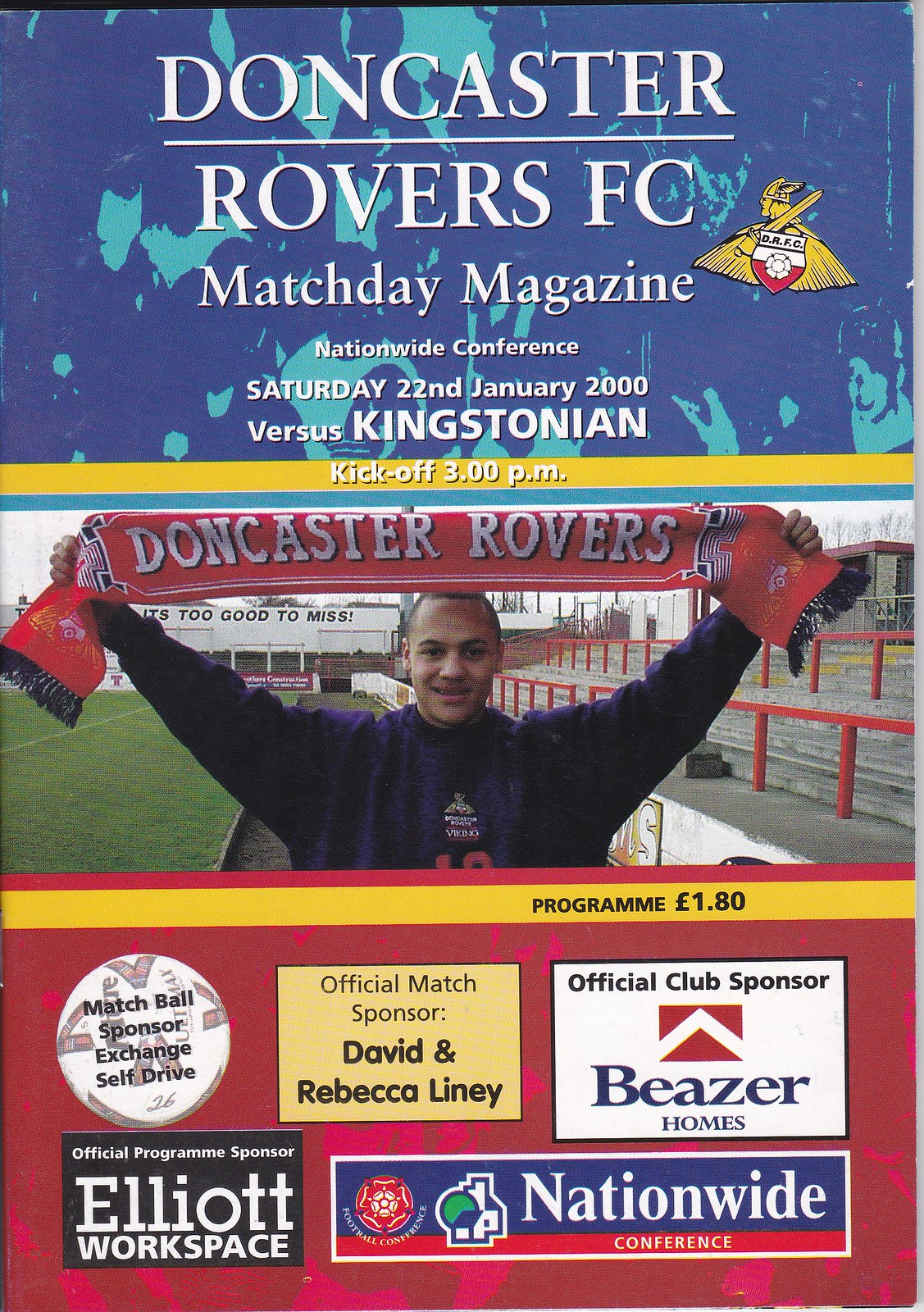The image depicts a magazine cover for a matchday program of Doncaster Rovers FC. At the top of the cover, white text on a blue background reads: "Doncaster Rovers FC Matchday Magazine, Nationwide Conference, Saturday 22nd January 2000, Versus Kingstonian, Kickoff 3.00 p.m." Below this, there's a photograph of a man standing by the field, holding a red scarf over his head that has "Doncaster Rovers" written on it in white letters, with small black fringes hanging off the scarf. The man is dressed in a blue, long-sleeved shirt and appears to be standing near stadium stands. Beneath the photograph, a horizontal yellow strip states "Program £1.80." At the bottom of the cover, logos and names of various sponsors are displayed, including Nationwide, Elliott Workspace, Tees for Homes, David and Rebecca, and Match Ball Sponsor Exchange Self Drive.